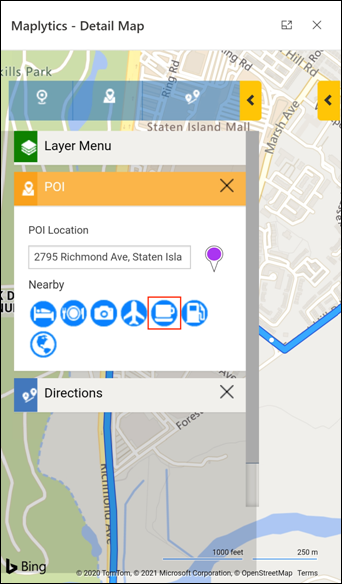This image is a detailed screenshot showcasing the interface of a mapping application. In the upper left corner, against a white header with bold black text, it states clearly "Maplytics Detail Map." Dominating the upper right section of the image is the map itself. Featured prominently on the map is a white informational box that labels a Point of Interest (POI) located at 2795 Richmond Avenue, Staten Island.

Overlaying the map are various icons representing amenities and services in the area, such as a bed symbolizing accommodation options, a fork, knife, and plate indicating dining establishments, a camera representing tourist attractions or photo spots, an airplane for transportation hubs, a cup for cafes, and a gas tank for fuel stations.

Above these icons, there is a header labeled "Layer Menu," which suggests additional customization options for the map's display. Positioned above this is a gray box, the purpose of which is not explicitly mentioned but might contain controls or additional information.

In the lower left corner of the map, the "B" logo for Bing is visible, indicating that Bing Maps is the map provider or source of the map data being displayed. The overall layout reflects a user-friendly interface with multiple functional elements to assist the viewer in navigating and locating key points of interest.